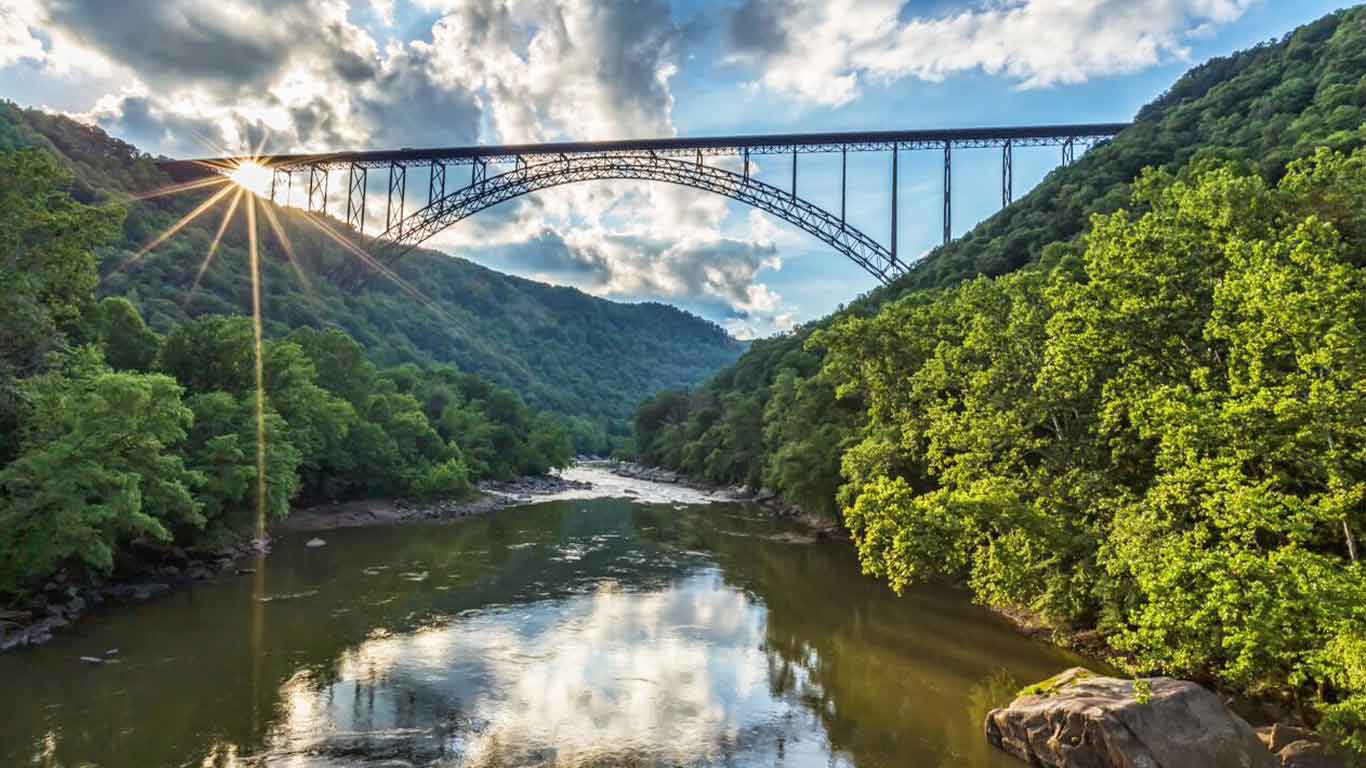The photograph captures a picturesque outdoor scene featuring a large black metal arched bridge spanning between two lush, green high hills, possibly even mountaintops. The scene is set towards evening, indicated by the soft, warm light and long shadows. The sun, positioned at the top left, shines down from above the hills, casting the bridge in silhouette. Below, a wide, shallow river with brownish water reflects the sky's white puffy clouds, and is flanked by rocks and dense, vibrant green foliage that grows darker deeper into the forest. The bright blue sky, adorned with scattered clouds, adds a serene backdrop to this natural landscape. The bridge, devoid of any visible people or structures, harmoniously connects the richly vegetated hillsides and traverses the serene river below, emphasizing the tranquil beauty of nature interrupted only by this man-made structure.